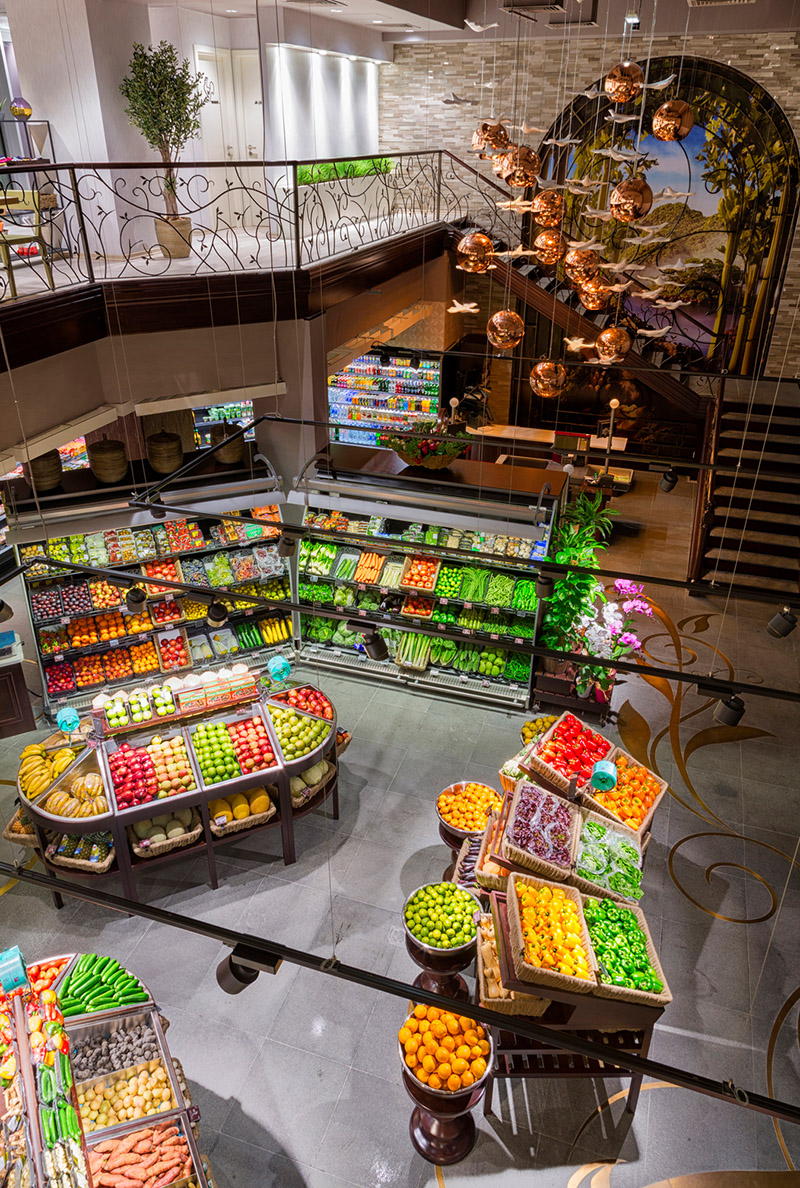The image captures an upscale, possibly multi-level market viewed from an elevated vantage point, about 20 feet in the air, giving a broad overview of the scene below. Various stands and displays are visible, laden with colorful produce such as apples, bananas, oranges, and bell peppers in both green and yellow hues, all arranged in smaller baskets and ornate setups. A prominent feature is a brassy, copper-colored mobile or chandelier hanging from the ceiling, adorned with globes and birds appearing to fly around them. To the right of the image, a metal railing, intricately patterned, leads up a stairway to a second level where additional displays and a tall potted plant stand against a gray and white brick backdrop with windows. Suspended from the ceiling in that area, another green plant hangs across the windows, contributing to the lush, vibrant ambiance of the space. The lower left of the frame also shows various types of candies in different colors, some in jars and boxes, further adding to the rich visual diversity of the market.